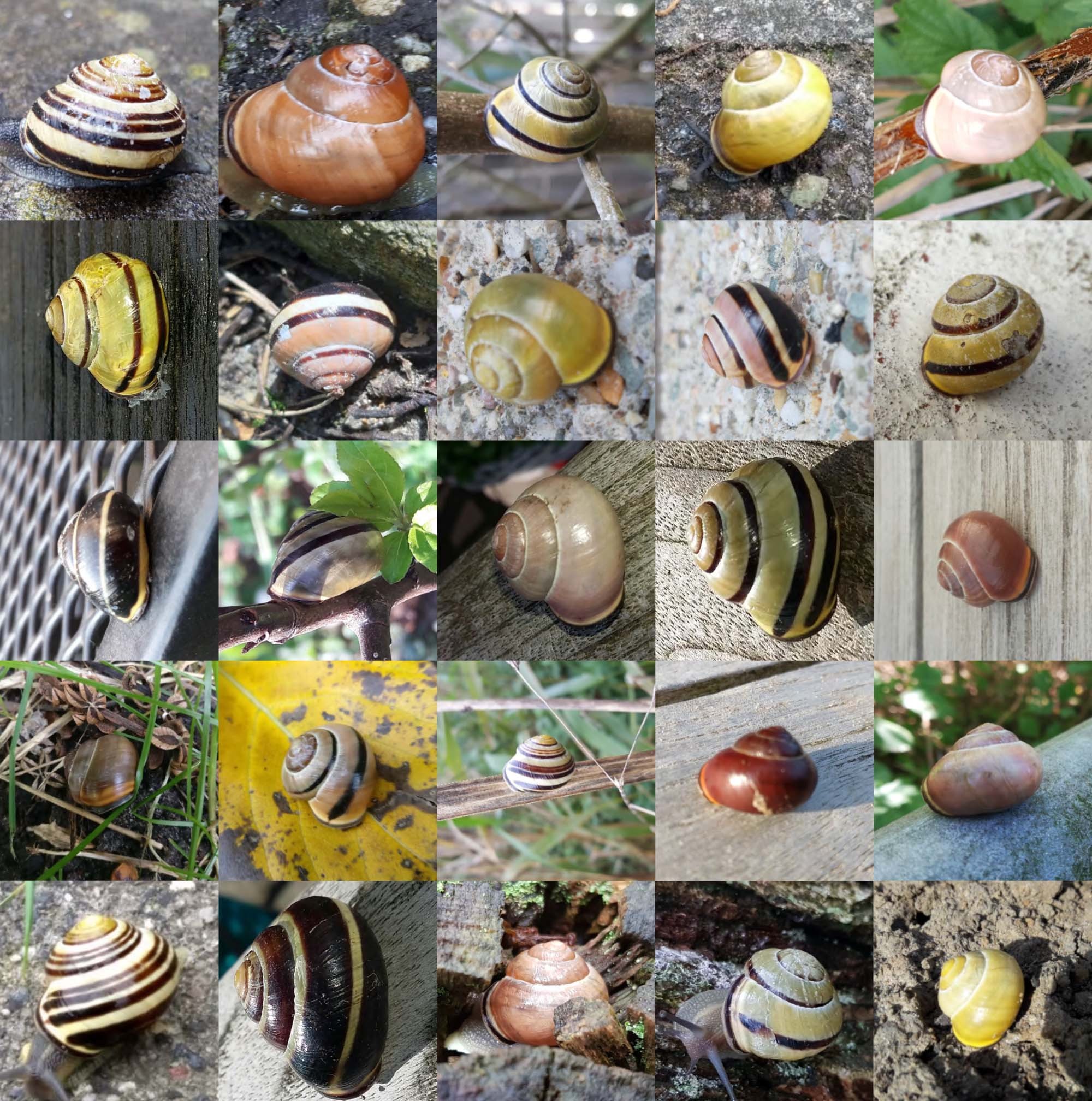The image is a captivating collage featuring 25 distinct snail photos arranged in a 5x5 grid. Each square showcases a unique snail with a variety of vibrant shell colors and patterns, ranging from yellow with black stripes to tan amber, and even brownish-red and pink hues. The snails are set against diverse backdrops, including pieces of wood, stone, leaves, grass, and dirt, highlighting the different environments where these snails can be found. The close-up shots emphasize the intricate details and uniqueness of each shell, making no two pictures identical. While some snails appear naturally in their habitats, others seem deliberately placed for a clearer view. Overall, the collage presents a visually appealing and detailed exploration of the fascinating diversity among snail shells.